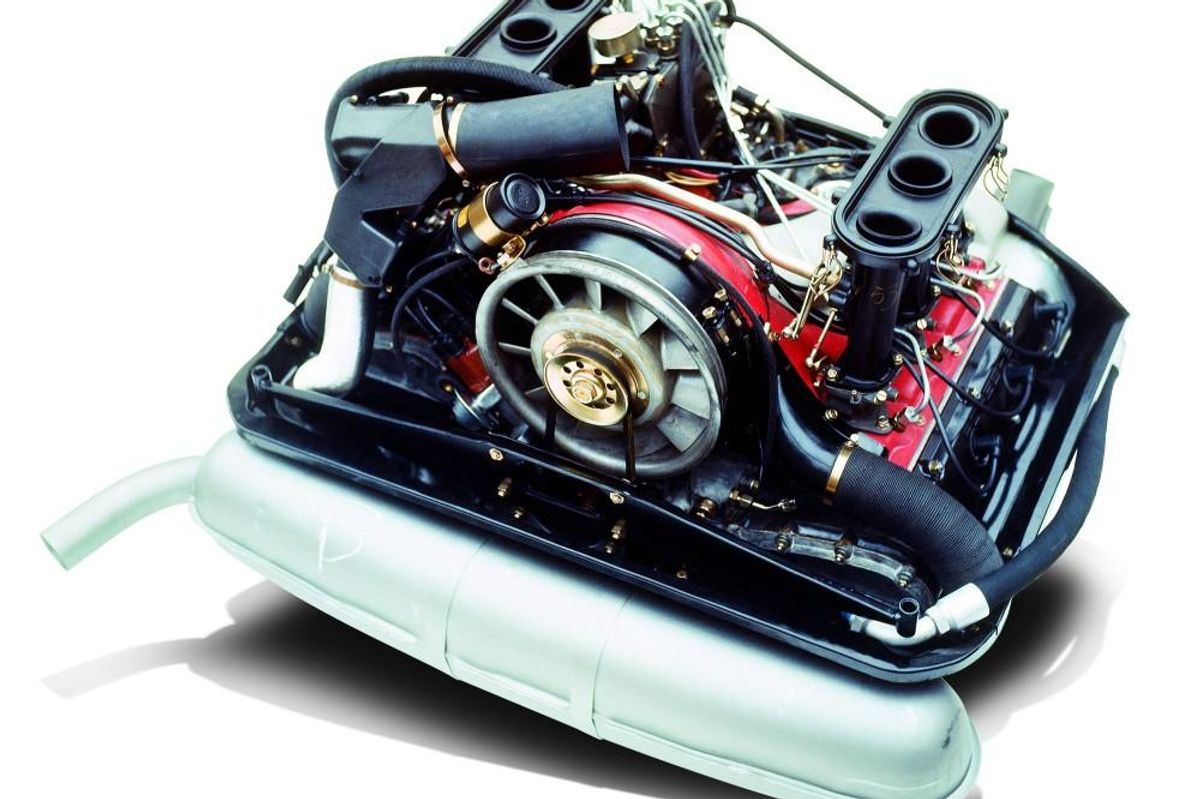This detailed color photograph showcases a close-up view of a complex mechanical component, which includes a variety of intricate parts. Central to the composition is a black engine-like piece featuring a moving fan connected to a belt. Adding to the complexity, an assembly of various black, white, and colorful wires snakes through the apparatus, leading to numerous screws and metal parts. Prominent within the image is a red compartment and silver elements, including a muffler-like section with attached piping. The entire setup appears meticulously clean and rests on a silvery-gray base, possibly indicating it's part of a larger appliance or machinery. With hints of orange, gold, and black details accentuating the equipment, the piece also includes a white background, giving it a crisp and clear presentation. This might be a component of a vacuum cleaner, an engine, or another sophisticated appliance.